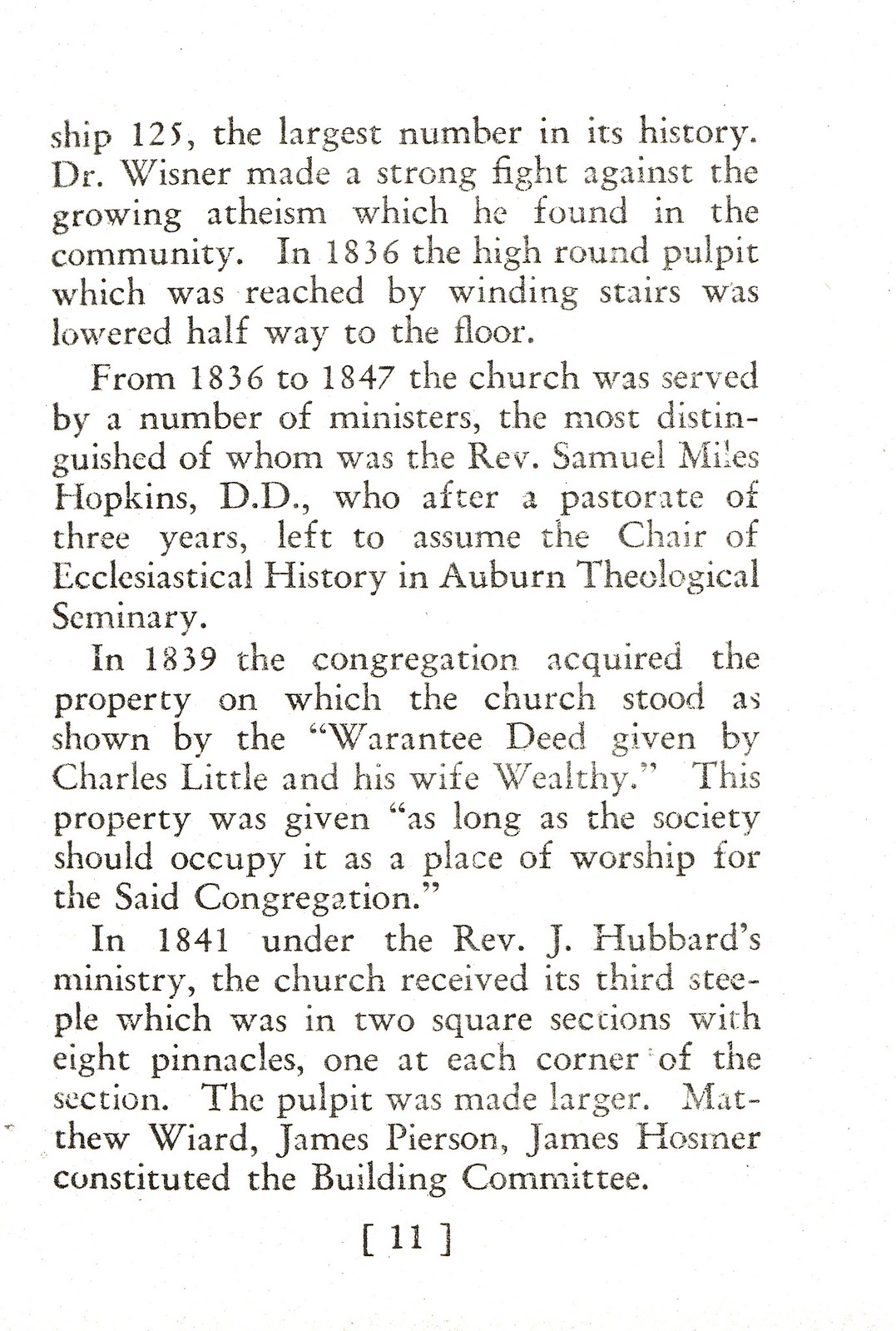The image displays a photocopy of a vertical rectangular page filled with text, set on a white background with black print. It appears to be a page from a book or old-timey newsletter, dating back to 1836. The text is divided into four paragraphs, detailing the contributions of Dr. Wiesner in fighting against growing atheism from 1836 to 1847. It chronicles the history of a church, including the lowering of its high round pulpit in 1836, the acquisition of its property through a warranty deed from Charles Little and his wife in 1839, and the addition of a third steeple under Reverend J. Hubbard’s ministry in 1841. The page also mentions several ministers, including Reverend Samuel Miles Hopkins, who left to join Auburn Theological Seminary, and building committee members Matthew Ward, Jim Pearson, and James Hosmer. The font style mimics that of an old newspaper, and the page number is marked "11" within brackets at the bottom.